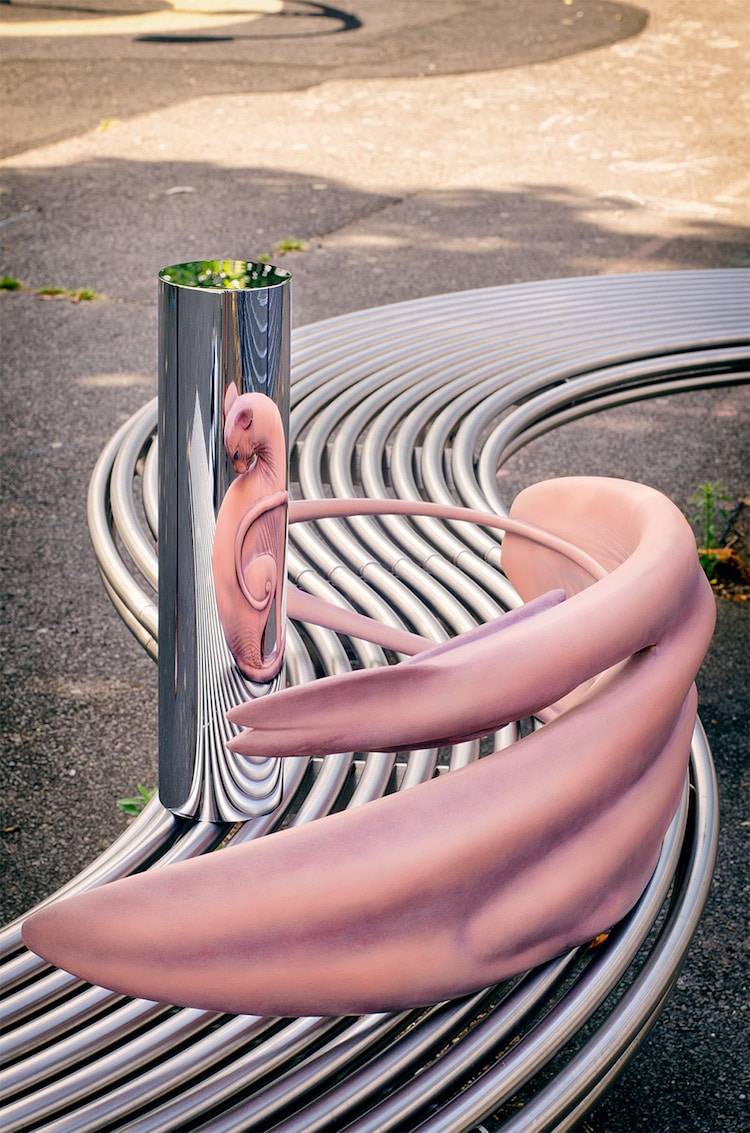The image depicts an art installation situated on an uneven, concrete surface with grass peeking through the cracks, hinting at a city sidewalk or driveway. At the foundation is a series of shiny, polished metal pipes that twist and curve in an S-shaped pattern. Sitting atop the left side of this metallic framework is a highly reflective chrome cylinder. Adjacent to it on the right side, a long, beige-pink-purple form resembling a stretched-out cat, actually a pink swirl, is visually transformed through an optical illusion. The cylinder's reflection astonishingly reveals the shape of a hairless cat, seemingly grooming itself, inside the metal pole. The bottom portion of the art piece includes floral elements contained within the piping, adding a touch of nature to the otherwise industrial aesthetic. The metal pipes create the illusion of a track, making the entire scene appear both intriguing and surreal.